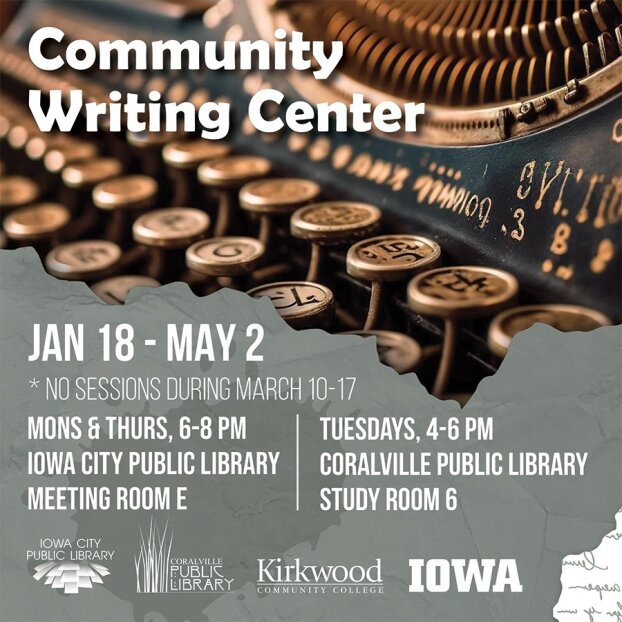The poster, promoting the Community Writing Center, features a captivating background image of an antique typewriter with copper-colored keys and intricate engravings on both the keys and the black-painted body of the machine. At the top, in bold white text, it states "Community Writing Center" followed by the schedule: "January 18th through May 2nd" with a note in smaller print, "No sessions during March 10th through 17th." The timing details beneath are listed as "Monday and Thursday, 6 to 8 p.m." at the "Iowa City Public Library, Meeting Room E" and "Tuesdays, 4 to 6 p.m." at the "Coralville Public Library, Study Room 6." The bottom of the poster displays logos for the Iowa City Public Library, Coralville Public Library, and Kirkwood Community College. A distinctive feature is a signature in black cursive on a ripped piece of white paper at the bottom right corner, adding a personalized touch to the polished design.